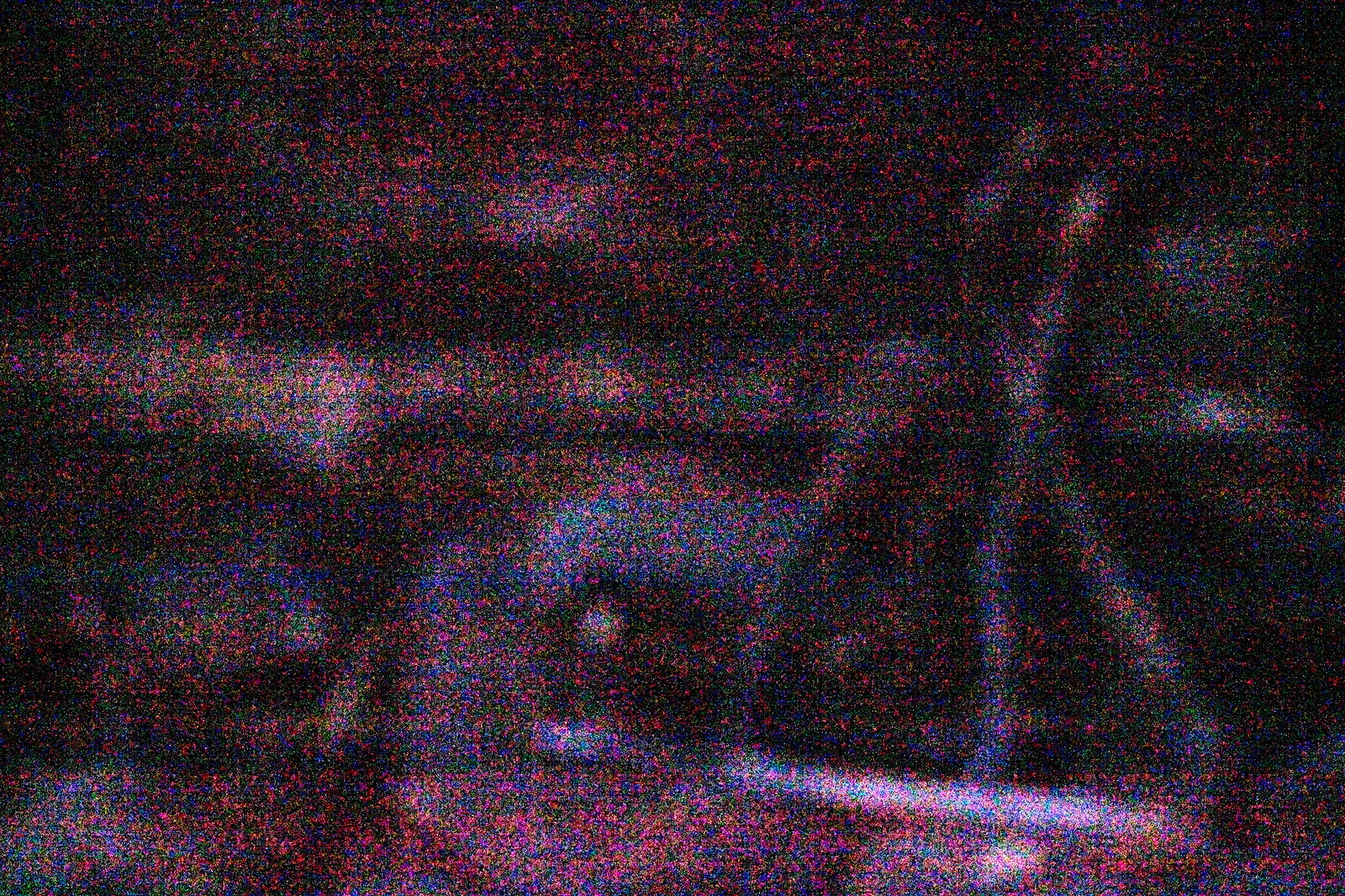A dark and grainy indoor photograph or digitally altered image characterized by a myriad of colored spots, including black, purple, green, yellow, and blue. The majority of the image is densely speckled with these tiny spots, making it challenging to discern whether the image is a photograph or digitally rendered. The lower half features some indistinct shapes; on the left, a form that vaguely resembles the profile of a head, while the center holds a round, slightly white shape that could be either another head or merely a circular form. Right of center, there are lines that seem to suggest the outline of a triangle or a similar geometric shape. Despite significantly increasing the contrast, the image remains ambiguous without any text or print, defined primarily by its mix of colors amidst the pervasive darkness.